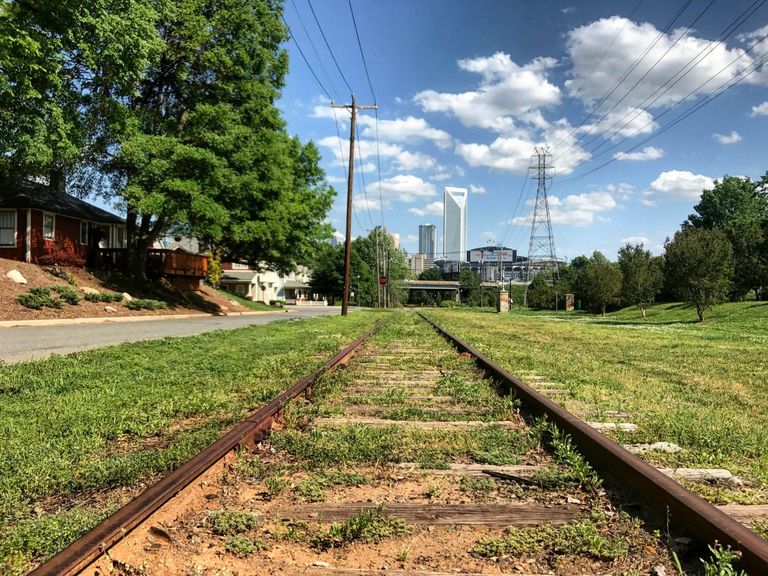This image captures a view from the vantage point of someone standing on railroad tracks looking towards a distant cityscape. The railroad tracks, which appear to still be intact and made of slightly rusty metal, are partially overgrown with grass and dirt, though the wooden ties remain visible. On either side of the tracks, there is well-kept grass, with a narrow asphalt road to the left that is bordered by more grass. A functional house stands to the left of the tracks, surrounded by large trees with green leaves, and further left, there is an area abundant with foliage.

In the distance, a city skyline comes into view, featuring distinct buildings including a very tall, white, triangular-shaped structure and a slightly shorter, black building to its left. There are numerous other tall buildings forming the backdrop.

Power lines stretch from the foreground all the way towards the city, with a large telephone pole on the left and an electrical pole or transformer on the right. There might be a stop sign or a railroad crossing gate visible along the tracks.

The sky above is a mix of blue with patches of fluffy white clouds, indicating a cloudy yet bright day. The overall scene is framed by natural greenery and urban elements, capturing a serene yet dynamic contrast between the rustic railway and the bustling city ahead.